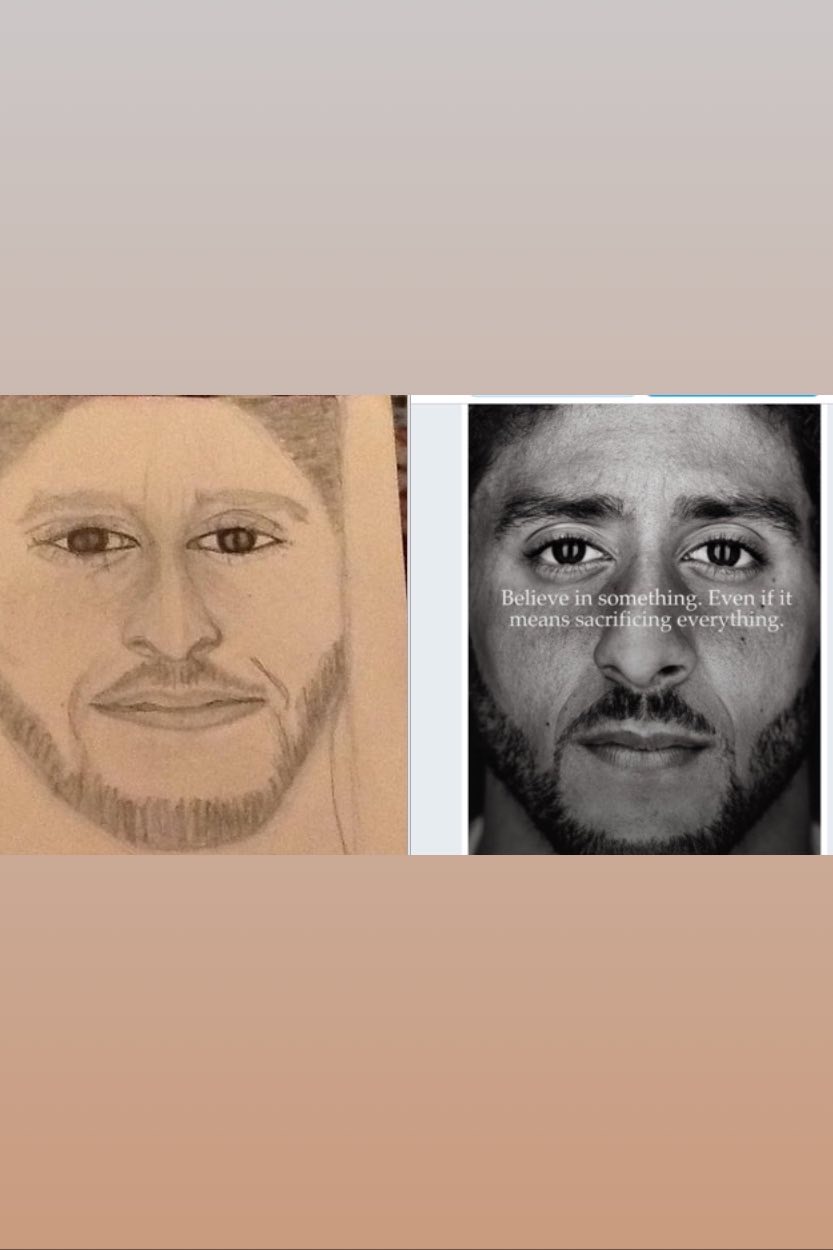Two images on a gray background depict Colin Kaepernick. To the right is a close-up, realistic photograph of his face, showcasing his dark eyes, dark eyebrows, shortly trimmed dark hair, and a neatly trimmed mustache and goatee. The quote "Believe in something, even if it means sacrificing everything" is printed in white text across the bridge of his nose. To the left is a pencil sketch, seemingly by an elementary school student, capturing Kaepernick's facial features with varying accuracy. The sketch portrays his dark eyes prominently, though with some inaccuracies in proportions and shading. Despite this, it evidently aims to represent Kaepernick.